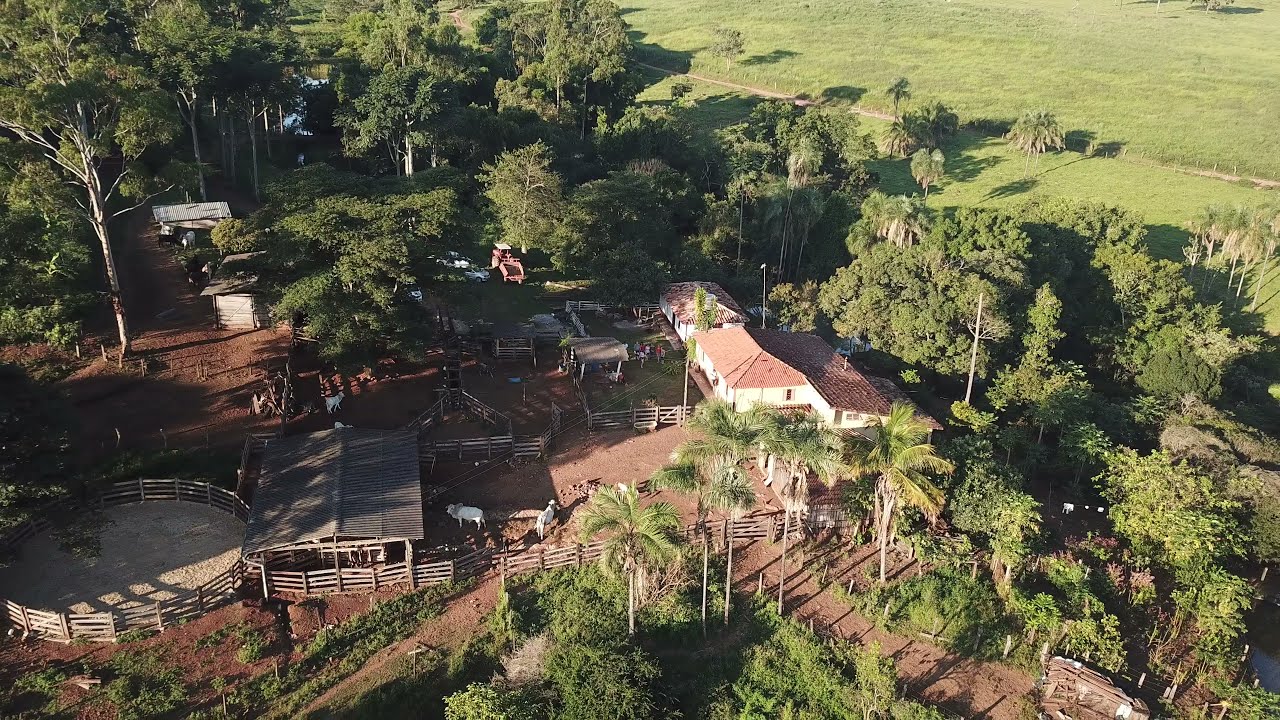The image depicts an aerial, daytime view of a sprawling ranch property. The eye-catching centerpiece is a white house with a prominent red roof situated on the right side. The landscape is characterized by plentiful dark red, clay-like dirt and numerous trees, including tall and short varieties, and notable palm trees. Surrounding the house, there are various outbuildings and structures, such as multiple sheds and barns.

Dominating the lower-left corner of the property is a circular exercise corral made of light wood fencing, distinctly horizontal in layout, ideal for equestrian activities. Adjacent to the corral is a barn, where at least two white cows or possibly other animals are fenced in. The ranch is crisscrossed by a dirt road that provides thorough access around the estate.

In the upper right-hand corner, a vast, well-manicured green field stretches out, slightly sloped upwards, suggesting an ideal pasture area. Not far from the main house, people are seen gathering in what appears to be a front yard. Additional details like a red tractor and various fenced enclosures further accentuate the functional and multifaceted nature of this picturesque ranch setting.